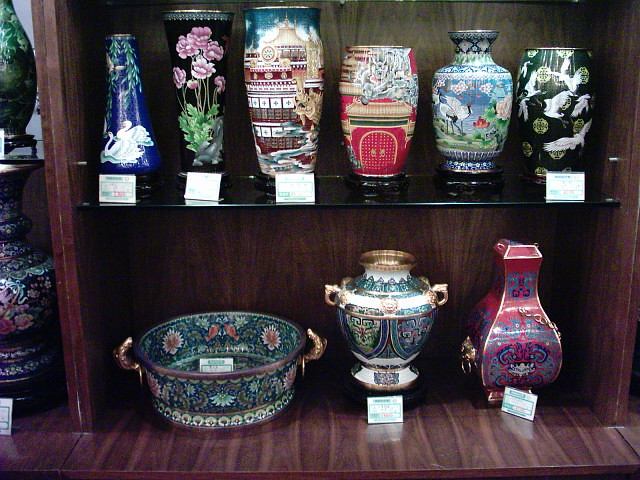The image depicts a museum-like display of assorted vases and urns within a dark, reddish wood grain cabinet, which features a single glass shelf at its midpoint. The cabinet showcases several intricately designed and possibly antique pieces, primarily of Asian origin, marked with small placards that might indicate their identity or price. On the top left, a striking black pot adorned with vivid green plants and pink flowers, displays a red-tagged price around a hundred dollars. Beside it stands a taller, thicker pot decorated with an elaborate temple and dragon motif—its red walls and yellow dragon head standing out. To the right, a slender-necked urn expands to a broader base, featuring red designs interlaced with light and dark blue elements. The display extends to the bottom right with a shallow bucket or pail with gold handles, while another section to the left holds additional vases—one notably adorned with stork imagery. The display's diverse shapes range from traditional vase styles to drum-like contours, all demonstrating a high degree of colorful, exotic artistry.